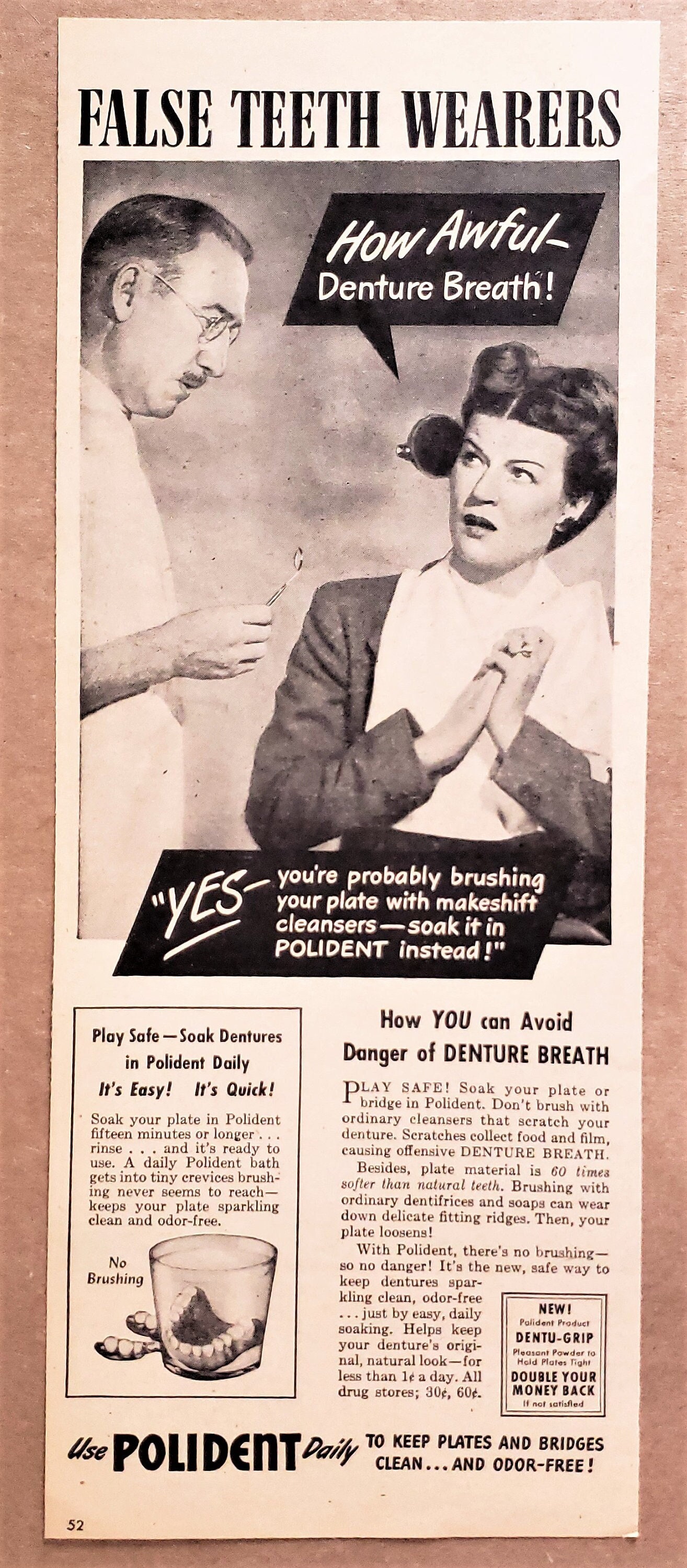This black and white vintage advertisement from the 1940s or 50s features a photograph set indoors, prominently depicting a dentist—a white man with circular glasses and a mustache—standing and gazing at a young woman in her 30s who is seated and wearing a gray jacket and dental bib. She gazes back at him with a distressed expression, exclaiming "How awful, denture breath!" The central theme of the ad revolves around combating denture breath. Text within black boxes emphasize the benefits of using Polydent: "Yes, you're probably brushing your plate with makeshift cleansers, soak it in Polydent instead," and "Play safe, soak dentures in Polydent daily. It's easy, it's quick."

The ad elaborates on the process of maintaining denture hygiene: "Soak your plate in Polydent for 15 minutes or longer, rinse, and it's ready to use. A daily Polydent bath gets into tiny crevices that brushing never seems to reach. It keeps your plate sparkling clean and odor-free. No brushing." Additionally, a small insert promotes a new Polydent product, Denture Grip, with a promise of "double your money back" if unsatisfied. The comprehensive promotional texts at the ad's bottom reiterate the importance of Polydent for keeping dentures clean and odor-free.

Enhancing the nostalgic feel, the photograph seems to be an aged newspaper article posted on a tan background, capturing the visual and textual appeal of mid-20th century advertising.